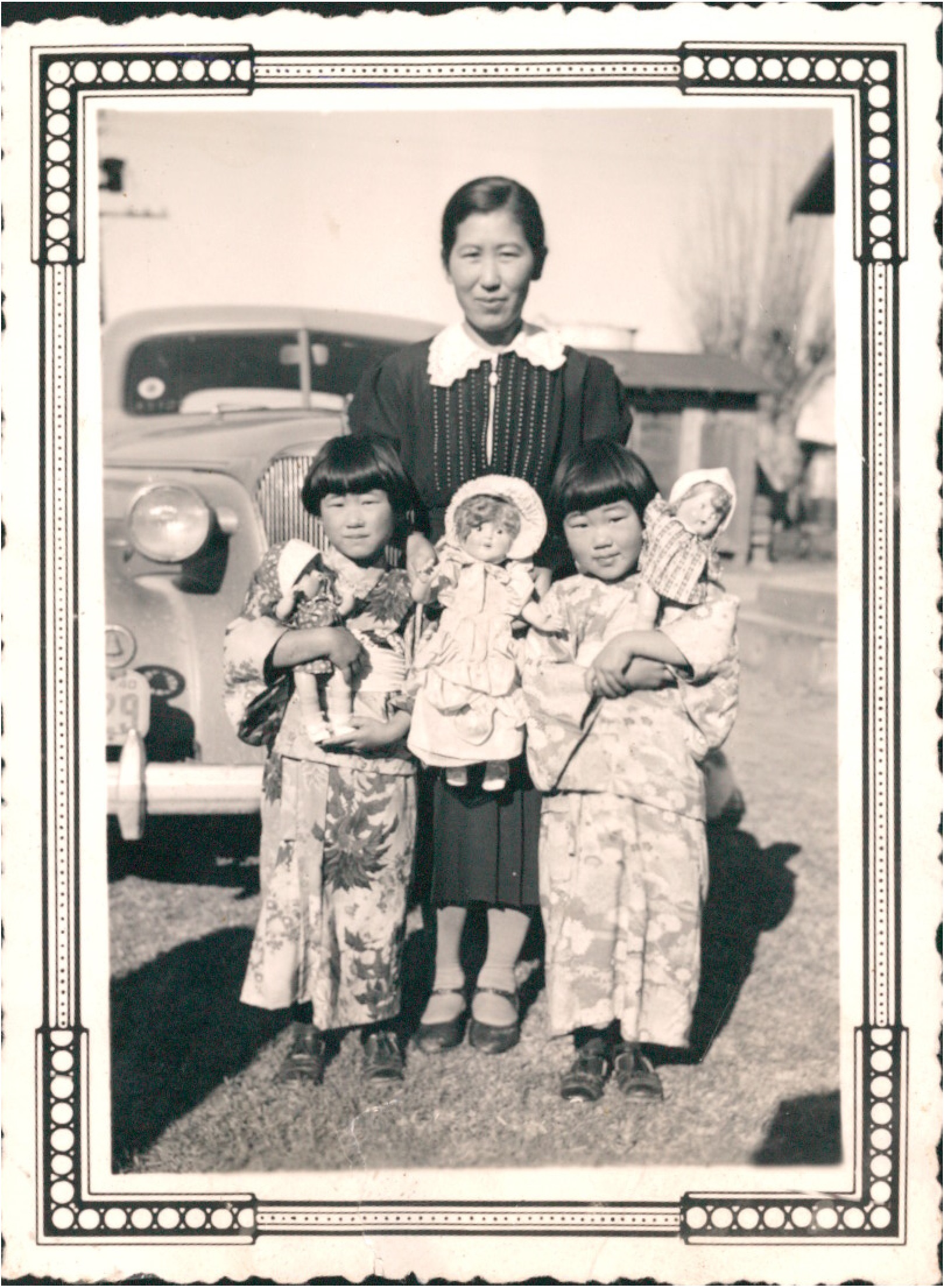In this black-and-white photo, an Asian woman stands outdoors with two children, both of Asian descent, centered in a garden setting. The woman, dressed in a long black dress with a white lace collar and black Mary Jane shoes, is holding a doll. Her hair is neatly tied up. Flanking her on either side, the children, who share similar hairstyles with black fringes, are dressed in camouflaged pantsuits and old-fashioned black shoes. Each child cradles a doll, creating a symmetrical and tender scene. Behind them, an antique car with a split windshield and a visible right taillight and bumper section adds to the sense of historical context. A tree without leaves and a shed can be seen in the background, suggesting a serene, rustic setting. The photo, framed with a geometric, ornate border, encapsulates a moment from a bygone era with intimate detail.